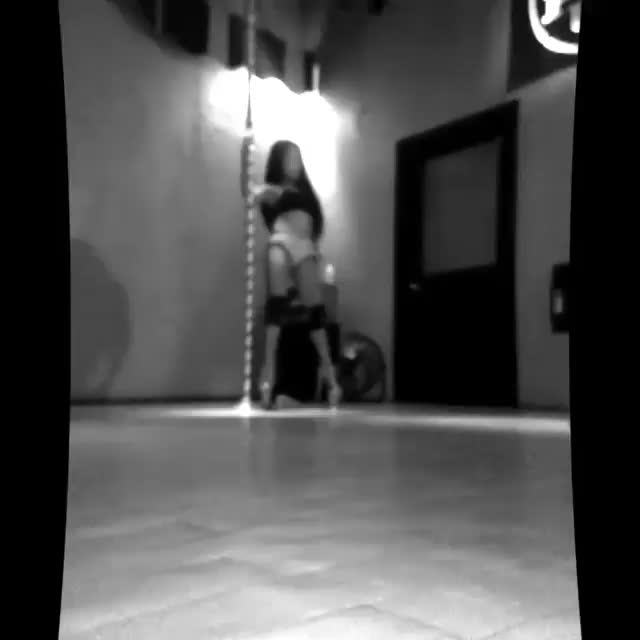The photograph is a grainy, black-and-white interior cell phone shot, featuring a solitary woman positioned next to a pole in the center-left of the image. Her attire is distinctly revealing: a dark brassiere-like top showcasing a bare midriff, paired with white panties and sleek stilettos. She sports long, dark hair that contrasts against her lighter complexion. Dark stripes adorn the pole she grips with her right hand, extending out of the frame vertically. 

The scene is sparse yet intense, with the concrete floor's gray surface empty save for the woman's striking presence and the spotlights casting concentrated beams of light. Three significant spotlight circles illuminate the area—two in the background and one in the foreground. The background is composed of uniformly gray walls, a large door with a bright brass handle, and an opaque window beside it. Though there's a spotlight above her marked by a blurred glow, her face and much of the surroundings are obscured due to the image's overall blurriness. The ambiance is dim and shadow-filled, hinting at a potentially evocative setting, further accentuated by the suggestive nature of her outfit and pose.